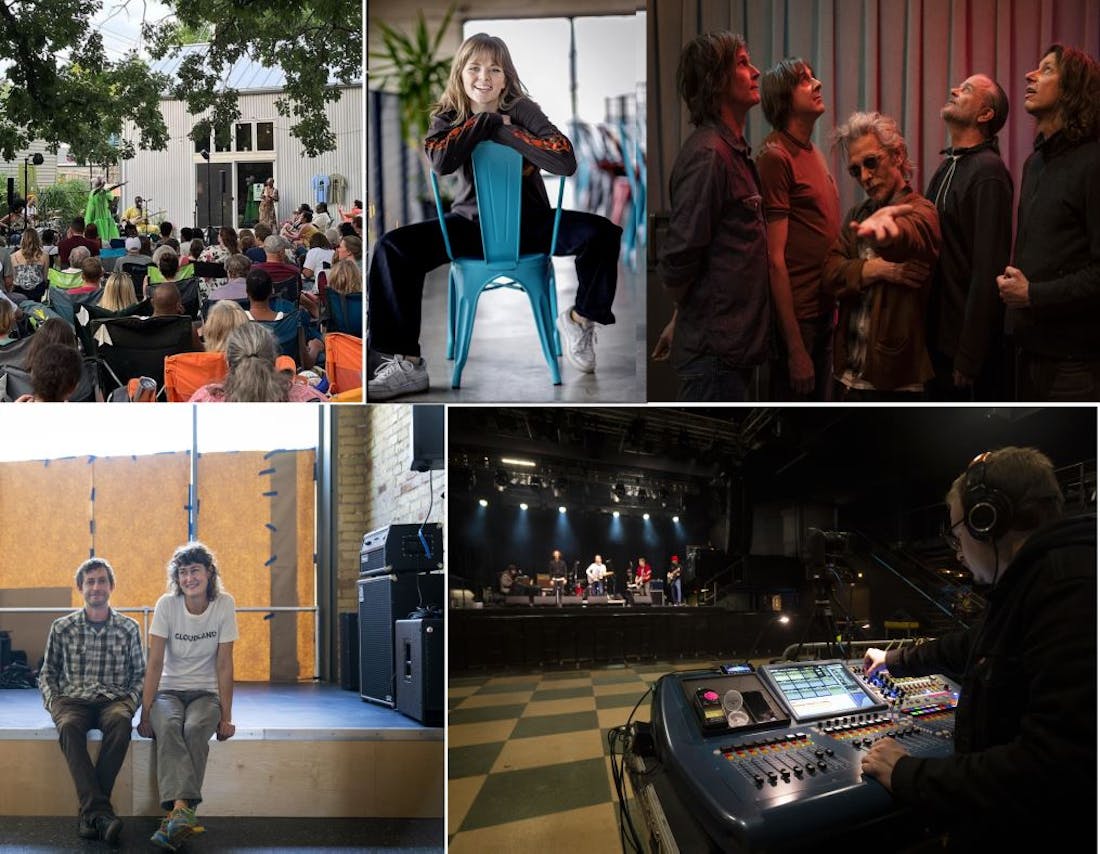This collage of five images presents scenes from what appears to be a music event. The upper left photo captures the backs of a diverse group of people sitting in colorful camping chairs (black, orange, teal), all turned towards a stage where a performer in a green costume stands in front of a building and under the shade of trees. Moving to the upper middle, a young blonde woman in black pants, white shoes, and a gray long-sleeve shirt with red accents sits backwards on a blue metal chair, smiling at the camera. The upper right image shows five older men who resemble a rock band. The central figure, with white hair and sunglasses, stands with his hand extended outwards, while the other four men (two on each side) gaze upwards. In the bottom left, two people— a man in a flannel shirt and dark khaki pants, and a woman with curly hair in a white t-shirt and khakis— sit on the edge of a stage next to some sound equipment, smiling at the camera. The bottom right photo features a sound engineer, wearing a hoodie and headphones, adjusting controls on a large blue soundboard, with a band performing on a brightly lit stage in the background.